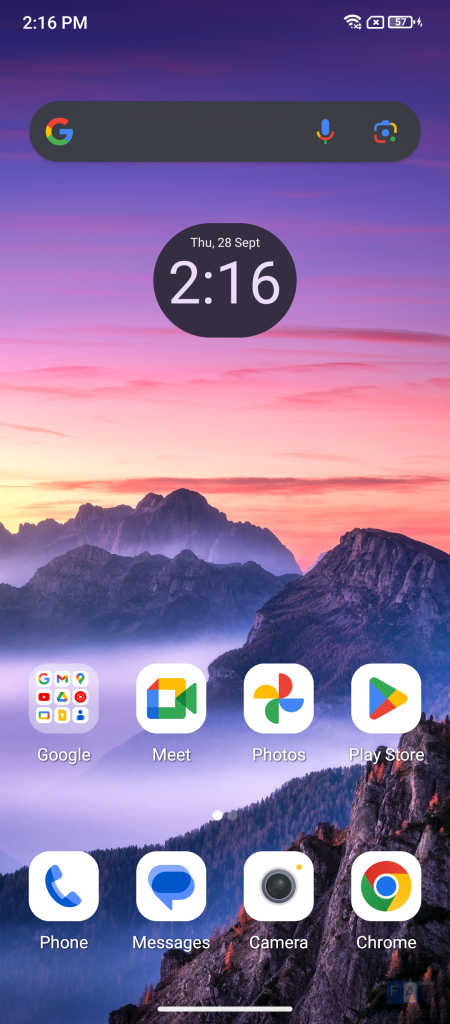A picture of a smartphone is set against a stunning natural background. The picturesque backdrop features a gradient sky transitioning from deep purple to vibrant pink and coral hues, which softly touch the peaks of distant mountains shrouded in misty clouds. The photo appears to be authentic and not digitally altered.

At the top of the phone's display, the time is noted as 2:16 PM, and the battery life is at a robust 97%. Below this, a Google search bar is prominently placed. The screen also reiterates the time and date: "Thursday, 28th of September, 2:16 PM," just in case the upper display wasn't noticed.

Embedded within the clouds beneath the mountain peaks are two rows of app icons. The first row includes a suite of Google applications: Google, Google Meet, Google Photos, and the Google Play Store. The second row features essential utilities: Phone, Messages, Camera, and Google Chrome—indicative of active online research. The well-organized display complements the serene yet captivating background, merging technology with natural beauty.